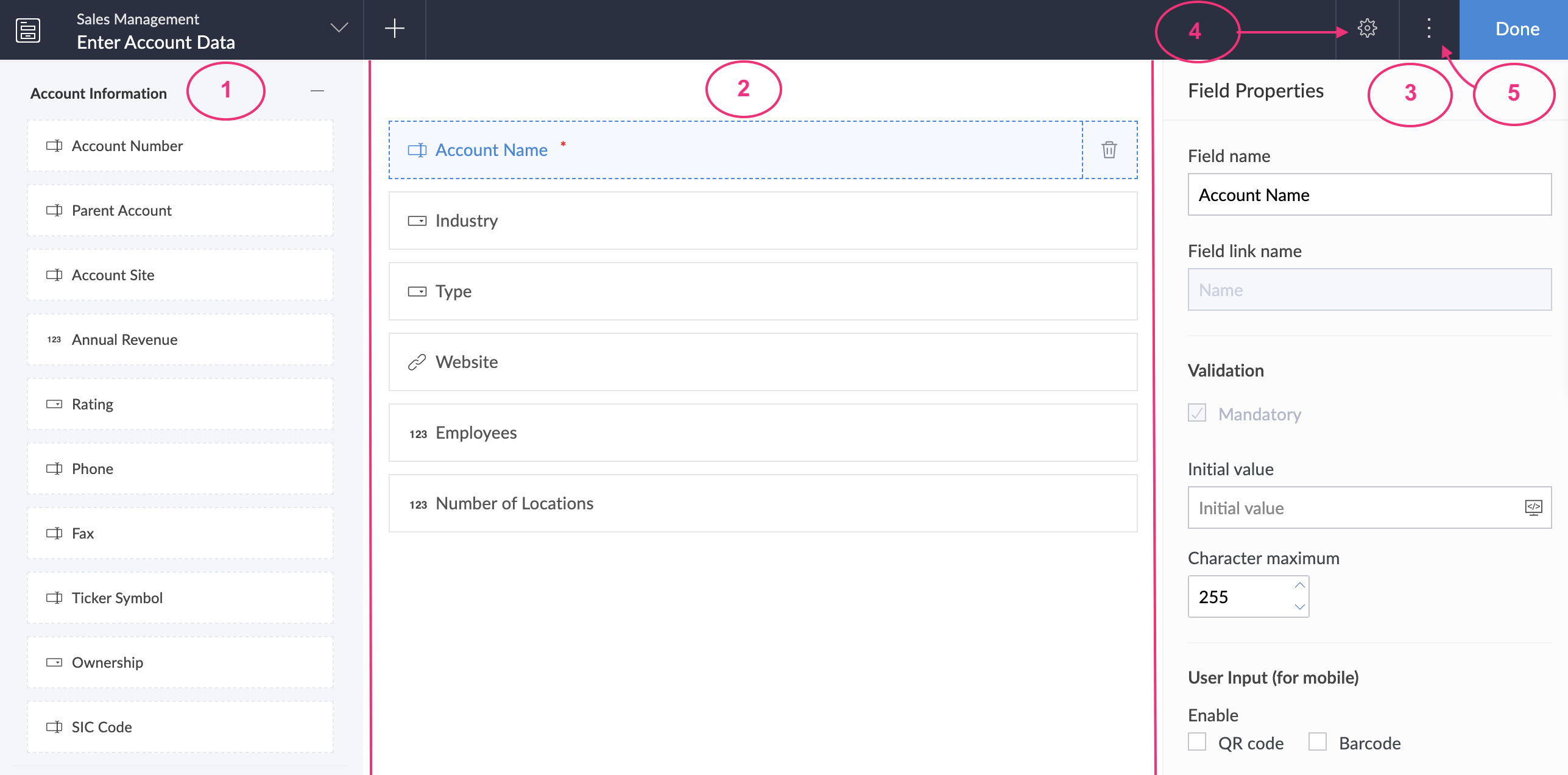The image displays a detailed annotation of a web application page used for entering account data, labeled with pink numbers enclosed in circles. Here's a breakdown of the annotated elements:

1. **Number 1 (Left Side - Account Information Section)**
   - Located on the left, this section is titled **"Account Information"**.
   - It contains fields such as:
     - Account Number
     - Parent Account
     - Account Site
     - Annual Revenue
     - Rating
     - Phone
     - Fax
     - Ticker Symbol
     - Ownership
     - SIC Code

2. **Number 2 (Center - Account Name Section)**
   - Positioned in the center, this section is titled **"Account Name"**.
   - The "Account Name" field has a blue dotted outline.
   - Below the account name field, additional fields include:
     - Industry
     - Type
     - Website
     - Employees
     - Number of Locations

3. **Number 3 (Right Side - Field Properties Section)**
   - On the right side, labeled **"Field Properties"**.
   - Under "Field Name," it lists "Account Name".
   - Below that, it provides options for "Field Name Link" and "Validation".
   - The "Mandatory" checkbox is checked.
   - "Initial Value" is indicated with a space for user input.
   - The maximum character limit is set to 255.
   - Additionally, under "User Input for Mobile," there are two unchecked options:
     - Enable QR Code
     - Enable Barcode

4. **Number 4 (Top Right - Settings)** 
   - Found on the top right corner of the page, denoted as **"Settings"**.

5. **Number 5 (Top Right - Options)**
   - Also located in the top right, labeled as **"Options"**.

**Header Section**
   - The page header has a dark background.
   - On the top left, it reads **"Sales Management"** with a directive to **"Enter Account Data"** accompanied by a drop-down icon. The text here is white.
   - Additional icons on the top left include:
     - A settings icon
     - A menu icon
     - A blue "Turn" button

This detailed view provides a comprehensive look at the structured layout and specific elements of the account data entry page within a sales management web application.